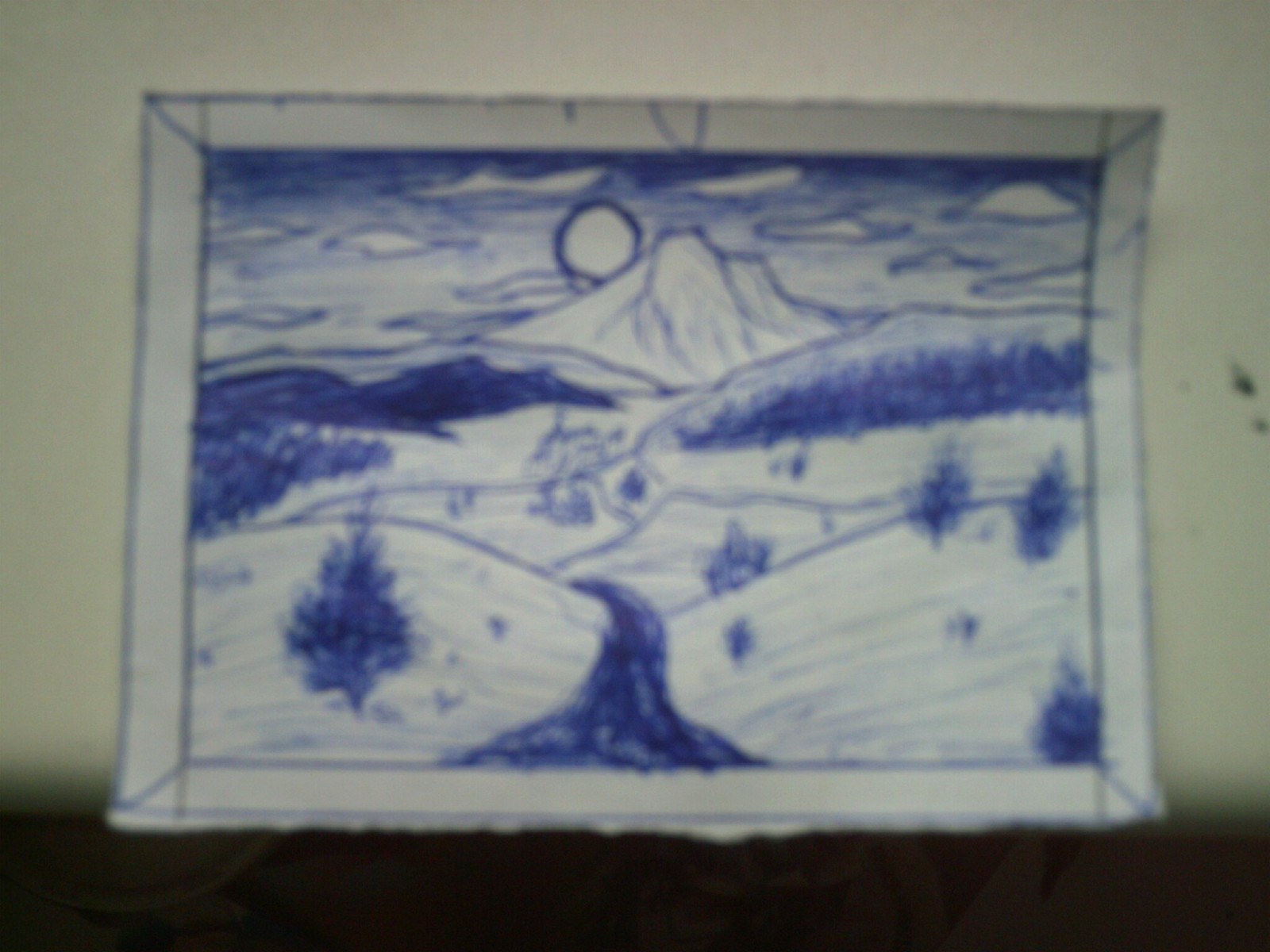This drawing, centered against a yellowish background, showcases a scenic landscape crafted with blue ink on a horizontally oriented piece of paper. The focal point is a winding road that traverses through a series of hills, each dotted with scattered trees. The hills recede into the distance, leading the viewer's eye to an outline of a building nestled in the background. Towering behind the building is a majestic, sunlit mountain, partially obscured by a few clouds drifting across the sky. On the left side of the composition, a shaded black mountain contrasts sharply with the taller, illuminated peak behind it. The road and some of the trees are also shaded, adding depth and texture to the scene. Beneath this artwork, a black line stretches horizontally, anchoring the piece within its yellowish frame.